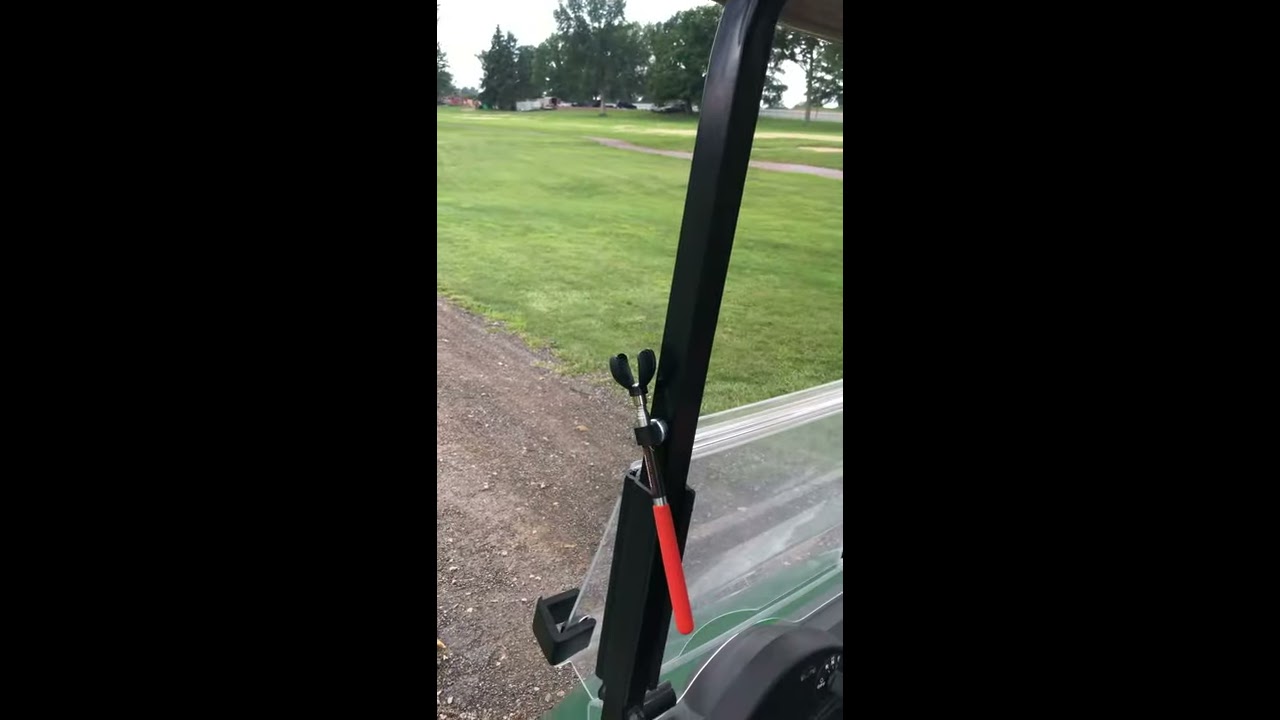The image depicts the left side of a moving golf cart, identifiable by its small steering wheel, mini windshield, and black metal rod supporting the roof. A noticeable attachment, which appears to be a red-handled tool resembling grabbers or a selfie stick, is affixed to the metal rod. The background showcases a green, open area that strongly resembles a golf course, featuring freshly cut grass, several trees, and two visible dirt trails – one running diagonally from the bottom left and another extending from the top right toward the center. The scene suggests the golf cart is in motion, capturing the serene landscape dominated by expanses of green fields and scattered trees.